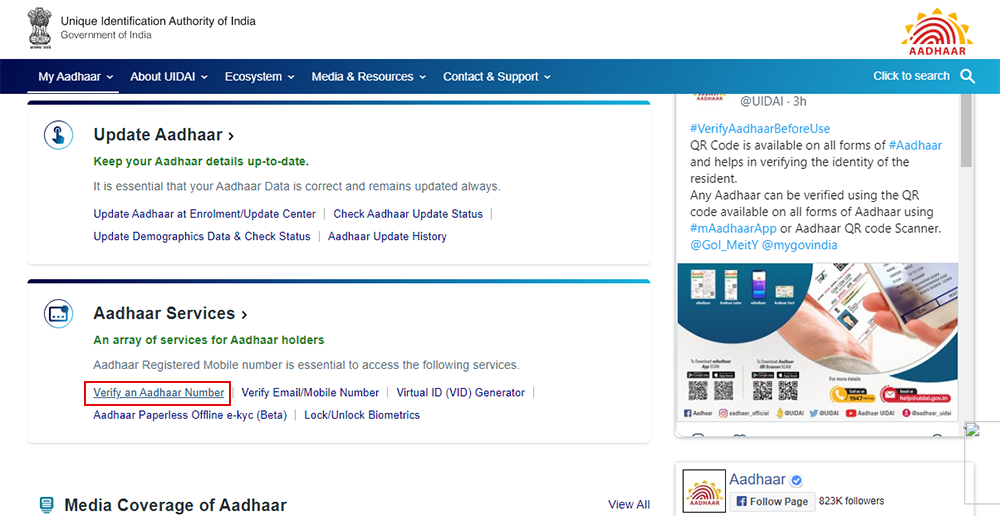A screenshot of the Unique Identification Authority of India (UIDAI) official website. This webpage, akin to the Social Security Administration in the United States, provides an array of services and information relevant to Indian residents. The site’s content is divided into handy sections covering various aspects such as media and resources, contact and support options, and organizational details. Key features include:

- Access to personal information and the ability to search for individual identification details.
- Comprehensive media coverage and social media links, including a Facebook follow option.
- Resources for understanding identification processes and resident identity verification.

The website facilitates essential updates, allowing users to modify their demographic data, view their update history, and track update status. Additional features enable email and phone number verification, creating a virtual ID, and engaging with paperless offline services—currently in beta. The option to unlock biometrics is also available.

The design features a white background with predominantly black and blue text, accented by green elements. An official government logo is prominently displayed on the left side, while a more vibrant red and yellow logo adds a touch of color and creativity to the right side of the screen.